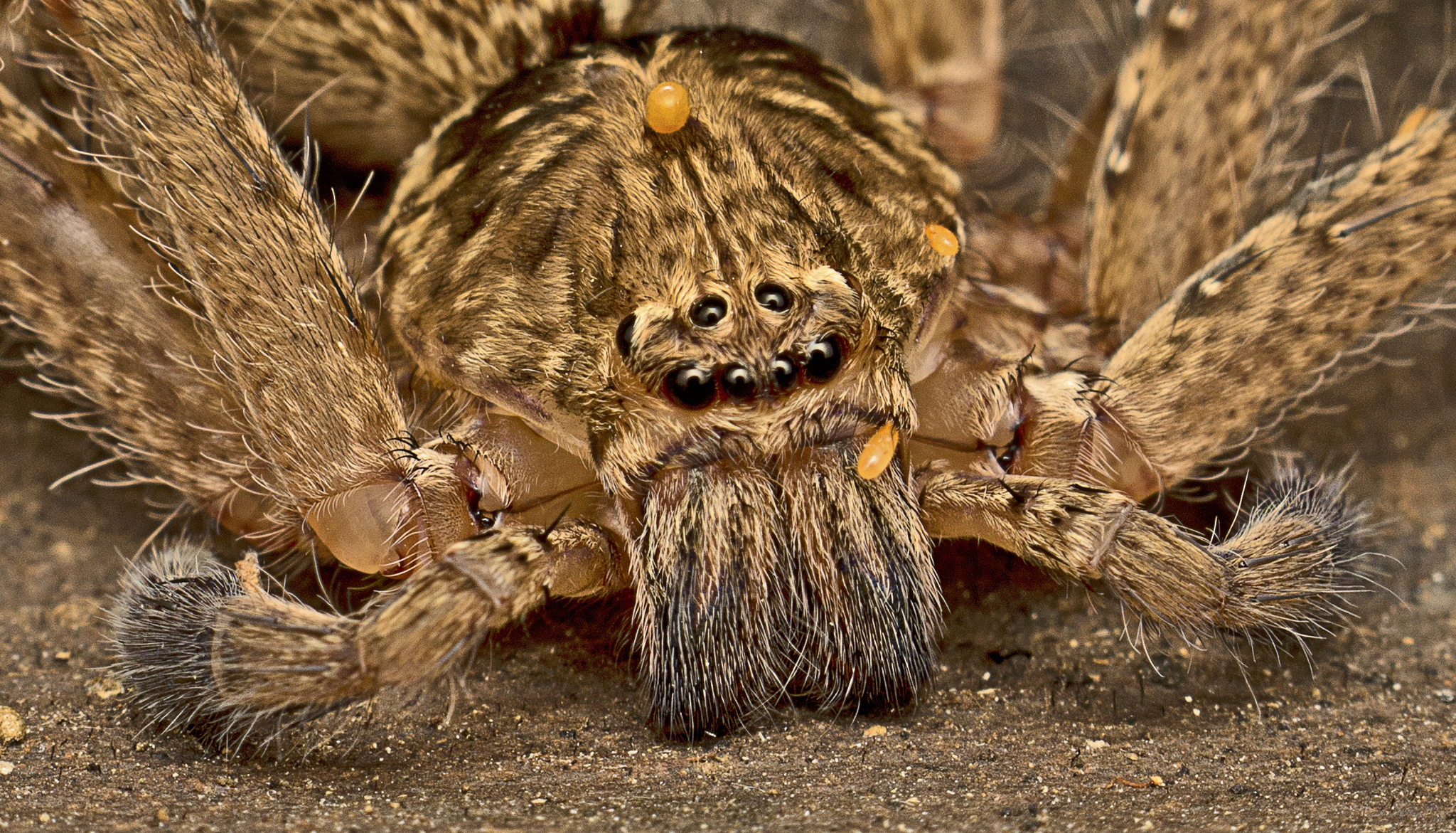This is a close-up photograph of a tarantula, taken from a head-on perspective, making it the central focus of the image. The tarantula, with its furry body, exhibits various shades of brown, tan, and black, along with hints of orange. It is positioned on a ground surface, possibly dirt, scattered with small pebbles, though it is uncertain if this setting is indoors or outdoors. 

The spider's eight legs, while not all fully visible, are covered in a mix of shorter and occasional longer white hairs, and they feature patterns of dark spots. Additionally, there are two prominent appendages near its mouth that resemble little brushes, which may not be legs but rather pedipalps used for sensing and feeding.

The tarantula's head features a notable "circle clamshell" structure with several small black eyes: two on the top, four at the front, and two on the sides, likely totaling eight eyes. Amidst its furry jaws and mandibles, which also appear covered in long hairs, are fangs concealed beneath the fur. There are also three distinctive orange, egg-shaped marks on its body – one on its head, one near the mouth, and one beside its right eye – which could be parts of its anatomy or remnants of something it encountered in its environment.